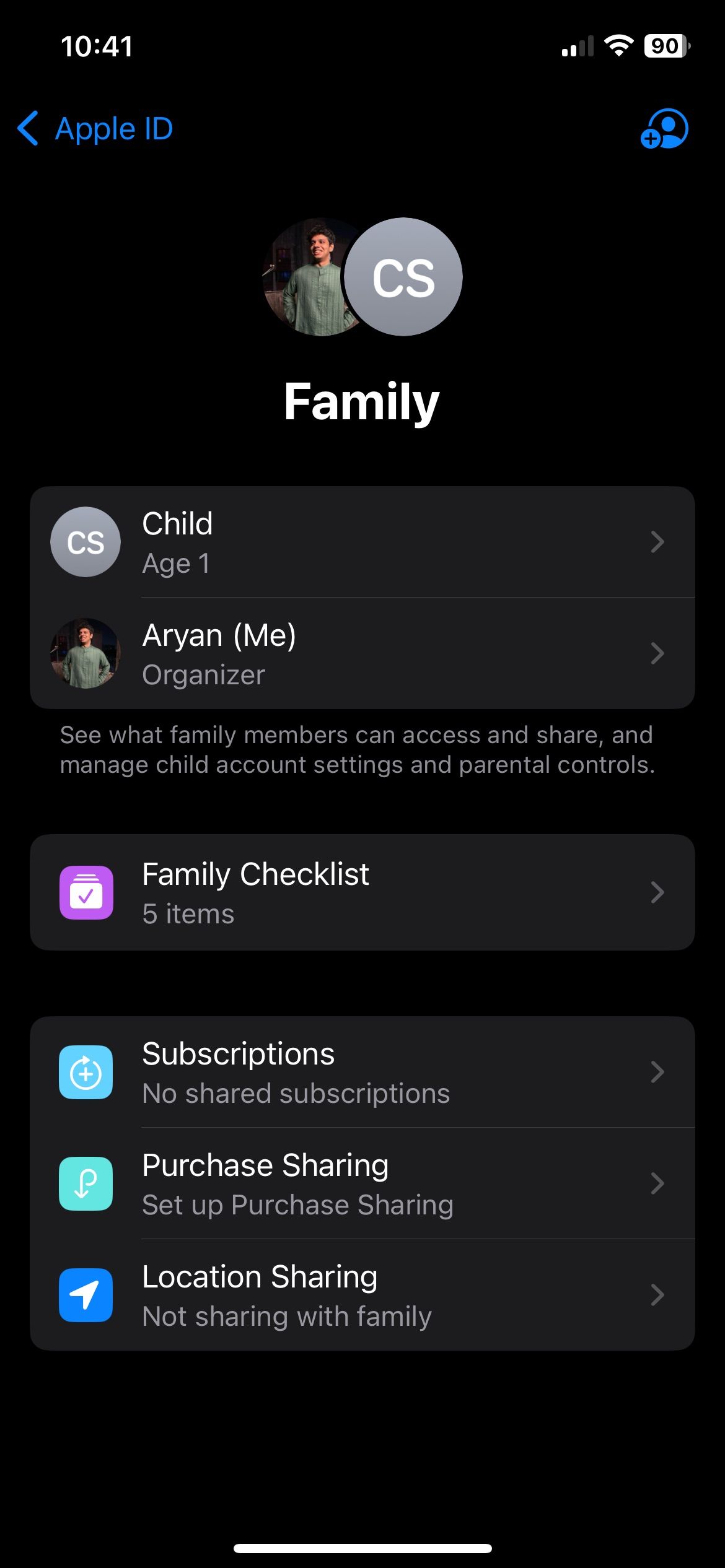This is an image of a phone screen displaying the Family Sharing section of an Apple ID. The background is completely black, and it is 10:41 AM. The battery is charged to 90% and the connection signal is strong.

At the top of the screen, "Apple ID" is highlighted in blue with a left-pointing arrow beside it. Below that, there is a circular icon featuring a person with a plus sign, representing a user profile. Adjacent to this icon is a gray circle containing the initials "CS" in white letters. This circle includes a small image of a person, who appears to be male and is wearing a green shirt.

Beneath the icon, the text "FAMILY" is displayed in capital letters and white font, indicating the family group section. The details of a child member are listed under this section, showing "Child, age 1." Further down, there is a gray circular image with "CS" inside it, followed by the name "Aaron (me)" indicating the user is the organizer of the family group.

The description below highlights various functions and settings:
- It mentions that you can see what family members can access and share, manage child account settings, and set parental controls.
- The "Family Checklist" section displays five items and is marked with a purple icon.
- Subscriptions are indicated by a blue icon.
- Purchase Sharing is shown with a teal icon.
- Location Sharing is represented with another blue icon.